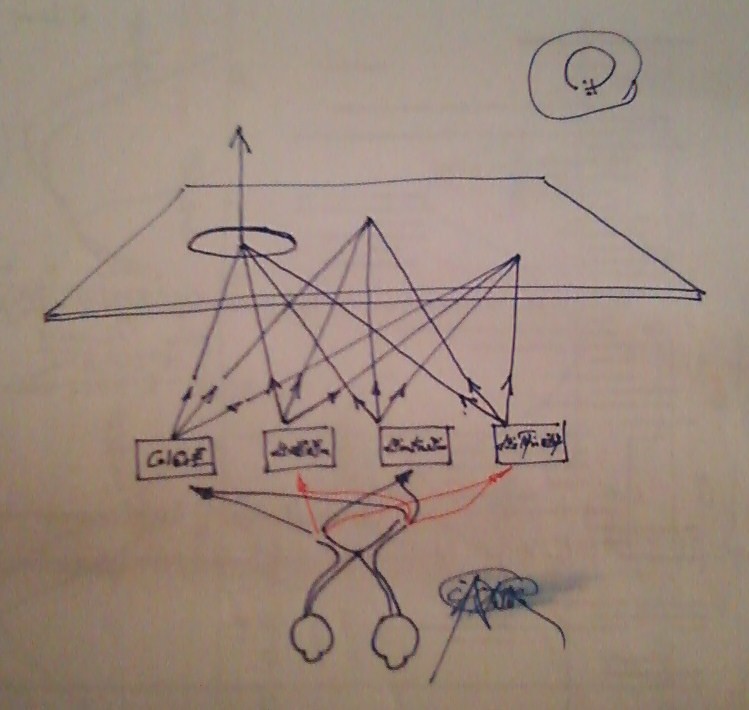The image showcases a detailed, ink-drawn scene set against a gray background. In the upper right corner, there are two concentric black circles that resemble a primitive drawing of a basketball hoop. Central to the composition is a large, elongated area dominated by a prominent circle through which a black arrow pierces upwards. Surrounding this central feature are four small squares, each containing letters and interconnected by an intricate web of arrows directing attention back to the central plane.

Beneath this primary area stands a distinct character, depicted with a large round body, slender legs, and disproportionately large feet, all rendered in black ink. This character is involved in the flow of the scene with one arrow extending from it and another returning to it. Highlighting this figure, there is a touch of red linking it to two separate blocks adorned with text. Additionally, a smaller character marked by blue and black hues appears at the scene's edge, also sporting thin legs, contributing to the overall complexity of the drawing.